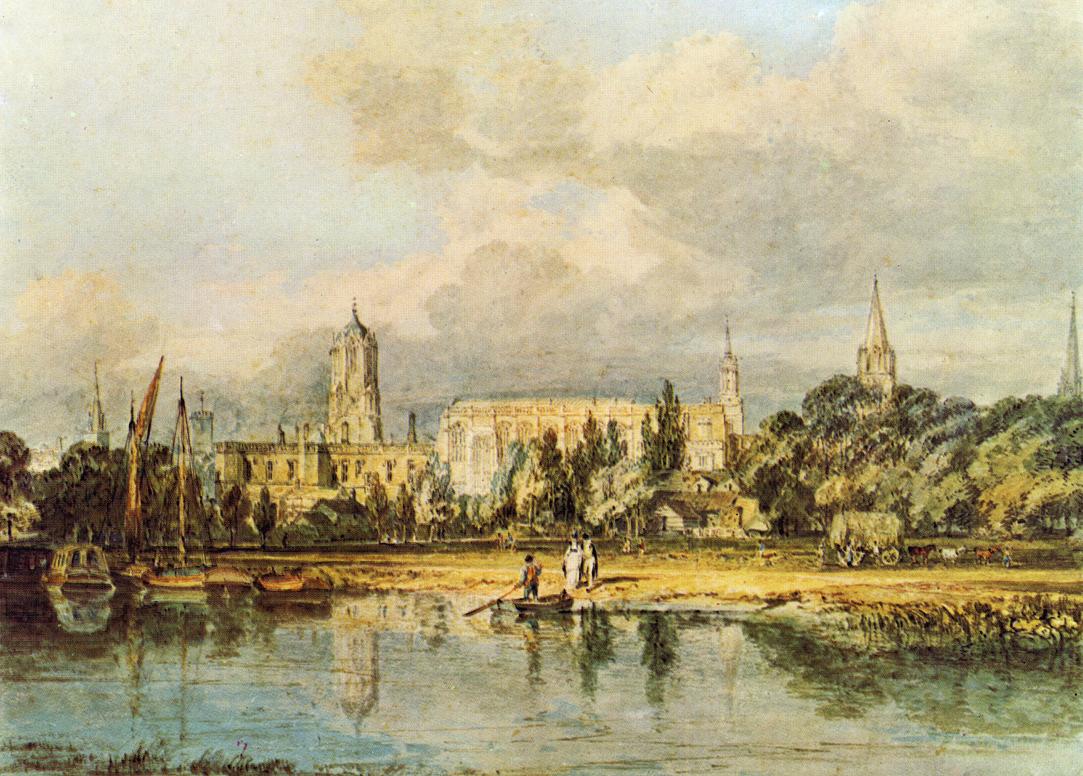This painting depicts a serene outdoor scene featuring a substantial, murky body of water that dominates the foreground. To the left, three vacant boats float idly near the water's edge. In the center, a solitary rowboat with one person inside is accompanied by two individuals standing on the distant shore, appearing to be either fishing or simply observing. The backdrop showcases a blend of natural and architectural elements: on the left, an old tan building with a pointed edifice resembling a church or cathedral, and to the right, amidst lush greenery and dense forest-like trees, stand three similarly pointed-topped structures. The sky above is overcast with clouds, suggesting it's a daylight scene, further enhanced by the painting's muted palette of light blue, gray, tan, yellow, black, and green hues. This visually compelling composition exudes a timeless quality, reminiscent of classical artwork one might encounter at an art exhibition.